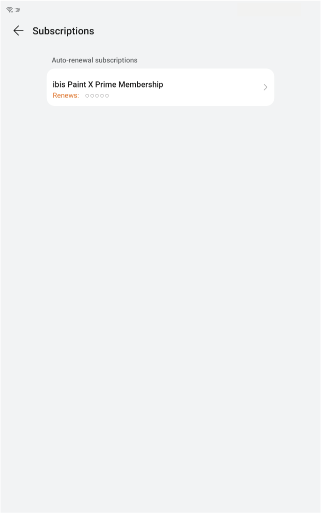Screenshot of Subscription Management Screen

The image depicts a straightforward subscription management screen with a focus on auto-renewal settings. At the top left corner, a back arrow allows users to navigate to the previous page. Below, the heading "Auto Renewal Subscriptions" is printed in a smaller font on a light gray background.

Dominating the center of the screen is a white, bubble-shaped box featuring subscription details. In bold, black letters within this box, it reads "IBIS Paint X Prime Membership." Directly beneath this, the term “Renews” appears in a gold-toned font, adjacent to which are several zeros displayed in a darker gray color, signifying the renewal status or date. The overall layout is minimalist, with a light gray background lending a clean and uncluttered appearance to the interface.